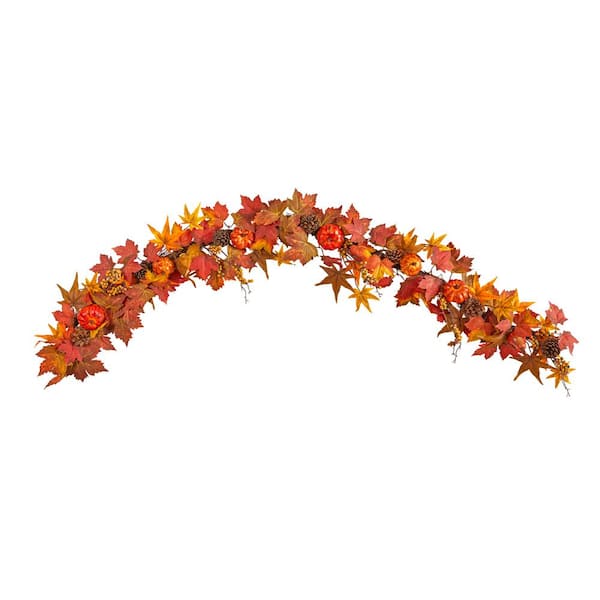This image features a decorative piece perfect for fall festivities, resembling a U-shaped or rainbow-bent wreath. The arrangement appears either as a wall hanging or centerpiece, richly adorned with quintessential autumn elements. A thin frame or possibly a wooden branch runs through the decoration, supporting an array of vibrant fall foliage and ornaments. Leaves in hues of red, orange, yellow, and brown—some shaped like stars and others like maple leaves—are interspersed throughout. Complementing the foliage are small, red fruit-like accents, possibly apples, and miniature pumpkins, enhancing its seasonal charm. Set against an entirely white background, the elegant display showcases this autumnal wreath in a way that makes it ideal for dinner events or festive gatherings, capturing the essence of the fall season.